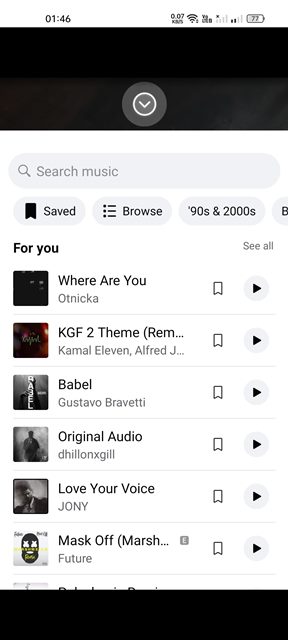The image depicts a cell phone screen displaying a music application interface. 

- **Top Bar:** 
   - **Time:** The upper left corner indicates the time as "01:46."
   - **Connectivity Icons:** The upper right corner features icons for wireless signal and cellular connection, along with a battery icon showing "77%" charge.

- **Main Interface Elements:**
   - **Notification Bar:** Below the top bar is a black rectangular box with a downward-pointing arrow.
   - **Search Box:** Directly below the notification bar is a search box with a magnifying glass icon and the prompt text "Search Music."

- **Navigation Tabs:**
   - **Saved:** Positioned on the far left.
   - **Browse:** Next to "Saved."
   - **90s and 2000s:** Located to the right of "Browse."

- **Recommendation Section:**
   - For You: The next line reads "For You" and "See All" on the far right.
   - **First Recommendation:** 
     - **Image:** A dark, unclear thumbnail image.
     - **Text:** "Where Are You," by Otnica.
     - **Play Button:** Located on the far right.
   - **Second Recommendation:**
     - **Image:** Another dark, difficult-to-discern thumbnail.
     - **Text:** "KGF2 Theme," by Kamal 11, Alfred J.
     - **Play Button:** On the far right.
   - **Third Recommendation:**
     - **Image:** Thumbnail with "B-A-B-E-L" text vertically.
     - **Text:** "Gustavo Breveti."
     - **Play Button:** On the far right.
   - **Fourth Recommendation:**
     - **Image:** Thumbnails featuring an indistinct figure.
     - **Text:** "Original Audio," by Dylan X. Gill.
     - **Play Button:** On the far right.
   - **Fifth Recommendation:**
     - **Image:** Thumbnail of a face, details unclear.
     - **Text:** "Love Your Voice," by Joni.
     - **Play Button:** On the far right.
   - **Sixth Recommendation:**
     - **Image:** Thumbnail of a face or mask with illegible text.
     - **Text:** "Mask Off," by Marsh Future.
     - **Play Button:** On the far right.

- **Bottom Bar:** A black rectangle spans the bottom of the page, possibly for navigation or additional controls.